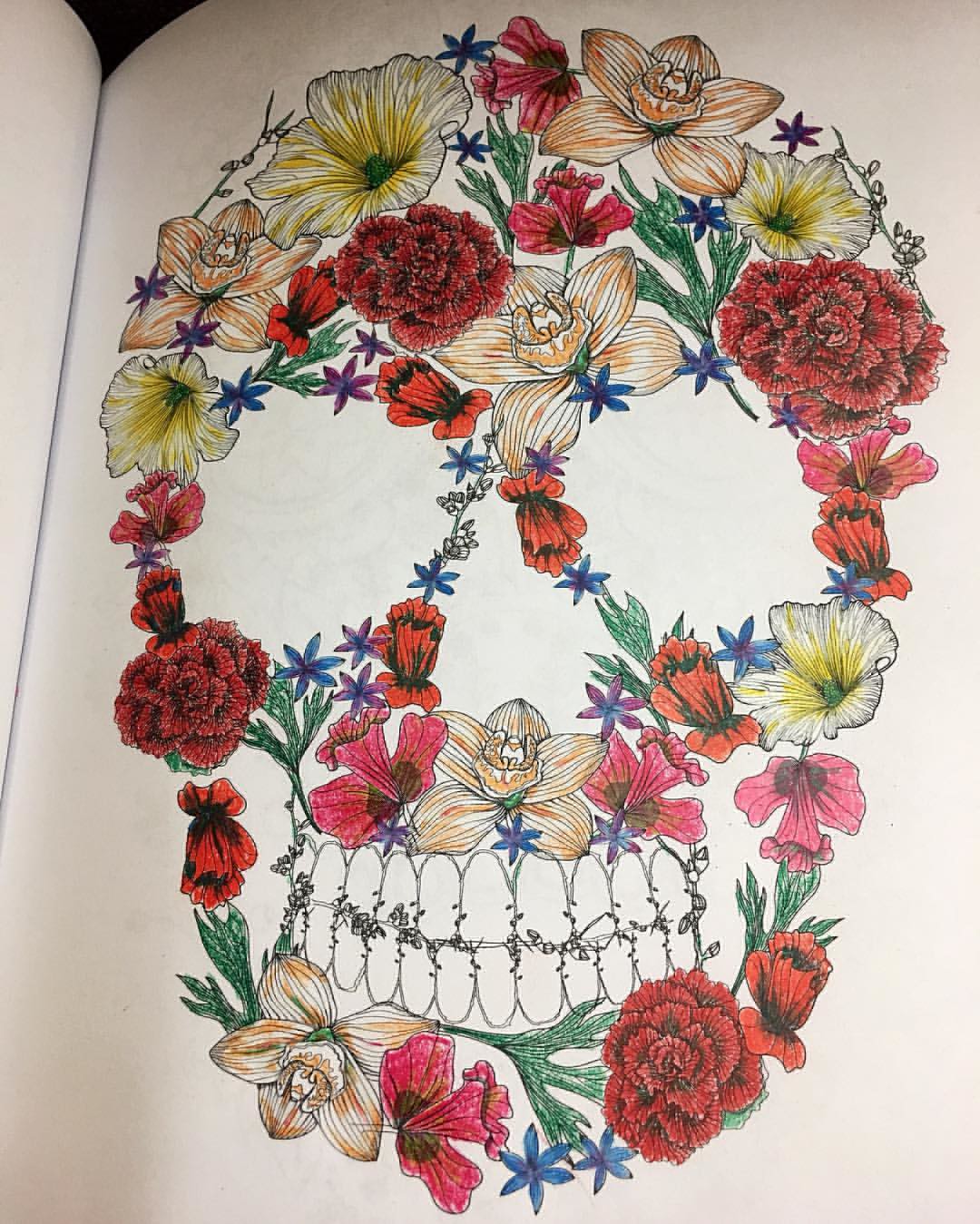This photograph captures a detailed piece of artwork created on a blank page of an artistic journal. The artwork is a vibrant illustration of a human skull, meticulously composed of various colorful flowers on plain white paper. The skull's outline and interior space are formed entirely by flowers of different varieties and hues, including red carnations, orange daisy-like flowers, yellow blooms, purple blossoms, and blue flowers, along with some green stems. 

The negative spaces precisely suggest the skull's eye sockets, nasal passage, and teeth. The eye sockets and nose are left as clear, white spaces surrounded by floral outlines, with the nose appearing as an empty triangle and the eyes as hollow ovals. The teeth are cleverly depicted using the stems and veins of the plants. The cheekbones are indicated by the arrangement of red and yellow flowers, giving structure to the face. 

A prominent beige flower is located centrally, below which the teeth are depicted with both the upper and lower jaw touching. Among the flowers are ones that resemble crosses with an extra line, adding intricate details to the image. The predominant color theme includes reds, yellows, and oranges, with a slight emphasis on red. Each element harmonizes to create a stunning, colorful representation of a skull, blending the macabre with natural beauty in an artistic and imaginative way.